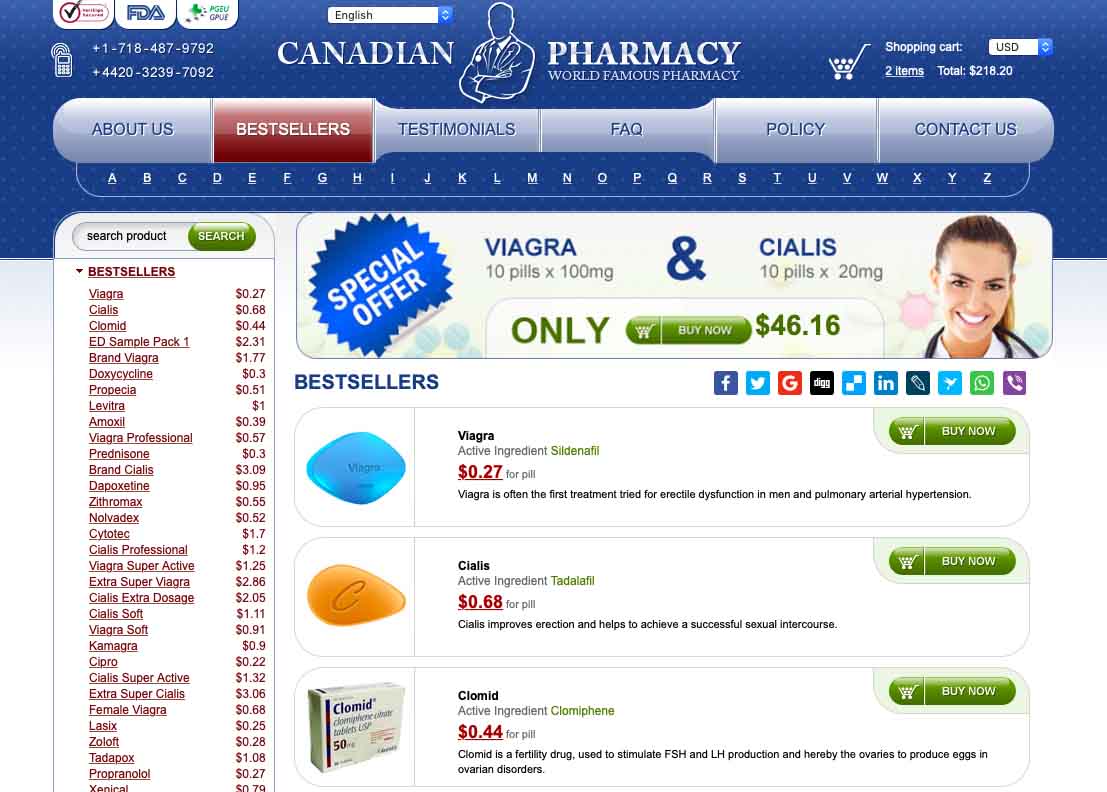This image is a cropped screenshot of the Canadian Pharmacy website. At the top center of the page is the "Canadian Pharmacy" logo, followed by the tagline "World Famous Pharmacy" in small, capitalized white letters situated to the right. Further right, in the upper corner, is a shopping cart icon accompanied by the label "Shopping Cart" in small white letters. Adjacent to this, a dropdown box set to USD appears, indicating the shopping currency. Below these elements, a summary notes "2 items, total $218.20."

On the top left, three partially cropped icons are visible, identified as 'Verified,' 'FDA,' and another unidentified icon. Directly underneath these icons are two telephone numbers paired with a small telephone clip art icon. Below this section, six grey bubble-shaped categories are listed: "About Us," "Best Sellers," "Testimonials," "FAQ," "Policy," and "Contact Us." The "Best Sellers" category is highlighted in red, indicating selection.

Underneath the categories lies a circular section featuring alphabetized links for further navigation. To the left, a white rectangular panel lists the best-selling items vertically, with the product names in red and prices displayed to the right. 

The center of the page begins with a banner announcing a special offer: "Viagra 10 Pills x 100mg" and "Cialis 10 Pills x 20mg" for $46.16, accompanied by a "Read By Now" button. Below this, the heading "Best Sellers" appears in large blue font, followed by three rectangular product boxes. Each box displays an image of the respective pill on the left, with the product name and description to the right. At the top right of each box is a green "Buy Now" button. The featured products include Viagra, Cialis, and Clomid.